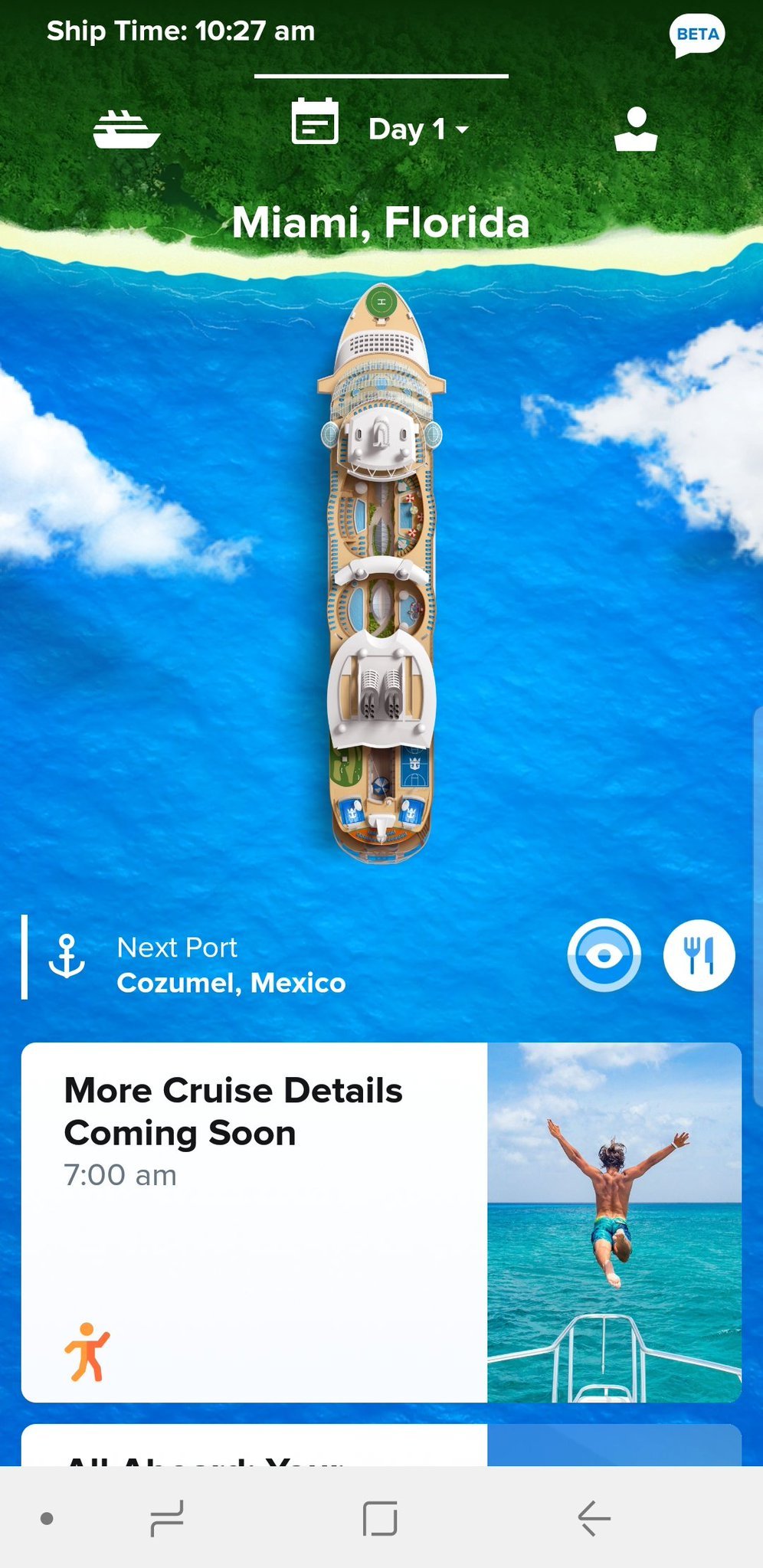A detailed screenshot from an Android beta mobile app designed for cruise line tours or scheduling, primarily for current cruise passengers. The interface is both functional and visually engaging. At the top, the app displays "Ship Time: 10:27 AM" and "Day One" with a dropdown menu for navigation. The top right corner is marked with a "Beta" label, indicating its testing phase.

Prominently featured is an illustrated top-down, bird's-eye view of a cruise ship on the water, complete with surrounding clouds. The ship's bow is docked against a sandy beach lined with green trees. This vivid illustration enhances the user's experience by offering a picturesque view of the ship’s location.

Below the illustration is an anchor icon followed by the text "Next Port: Cozumel, Mexico." Adjacent to this are two icons: one resembling an eyeball, likely indicating sight-seeing information, and another of a fork and knife, hinting at dining options or recommendations.

Further down, a message box reads "More cruise details coming soon, 7 AM," accompanied by an image of a person joyfully diving off the front of a small boat into crystal-clear blue water. The interface includes icons of a boat and a person, making it user-friendly and intuitive for cruise passengers to navigate their journey.